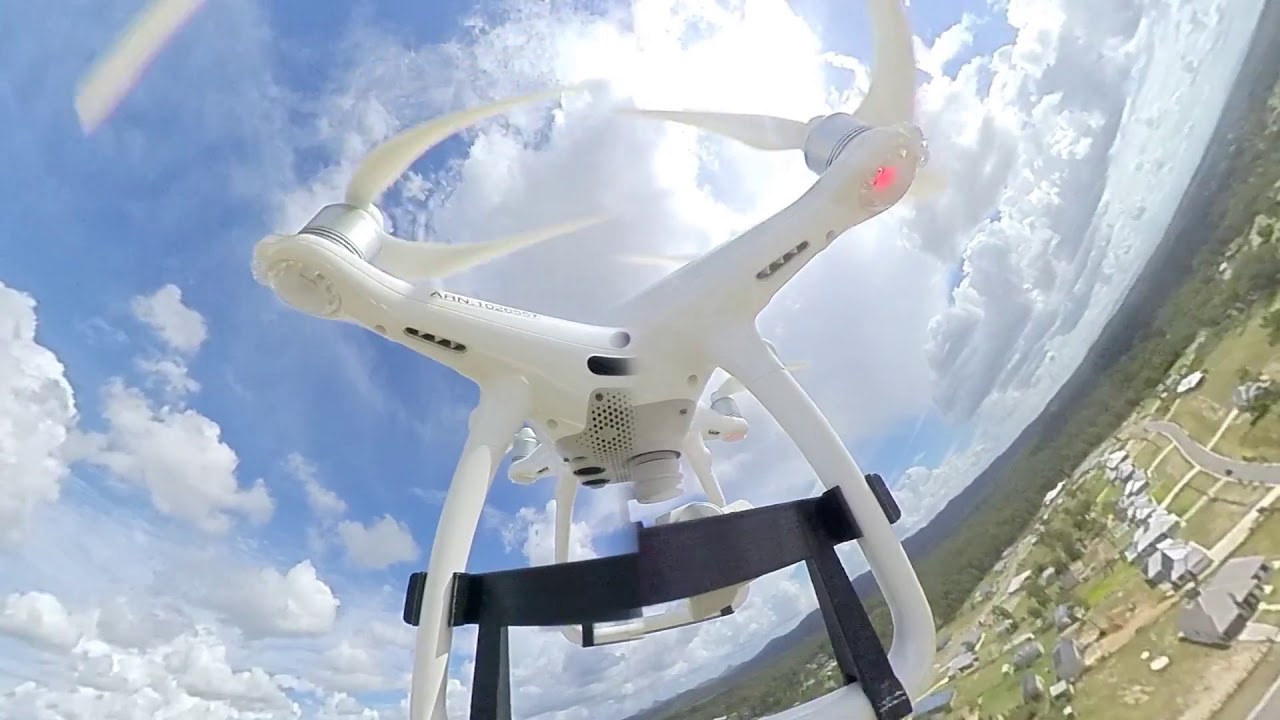The image captures a DJ Maverick drone mid-flight over a sprawling suburban landscape on a partly cloudy day. The white, star-shaped drone with four hovering rotors and a sturdy, hard plastic construction is prominently centered in the frame. It features black attachments, including what appears to be a custom 3D-printed holder securing the camera, and exhaust vents. The viewpoint of the image is an aerial shot from the drone's vantage, angled slightly to the right. Below, the scene reveals a densely-packed residential area with numerous houses and winding asphalt roads, interspersed with lush green trees. In the distance, a mountainous range stretches under a blue sky dotted with fluffy white clouds. The vivid colors in the scene—various shades of blue, white, gray, pink, black, and green—enhance the detailed and expansive view.